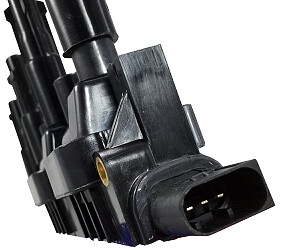This image features an ignition coil for a 2005 Mercedes Class A, designed for a 1.6L 8-volt engine. The device, predominantly black with some lighter shades, combines metal and plastic components. At the top, it has a cylindrical connector, angled slightly, with a round cylinder intersecting a larger one beneath it. This sits above a square base, from which a triangular support extends. The right side of the device showcases three metal prongs, indicating where connections are made, while the lower right corner includes indistinct white text or buttons, suggesting some kind of descriptive labeling. The entire assembly, with four short handles on its sides and additional protrusions, is presented at a slight angle, reminiscent of a catalog display.